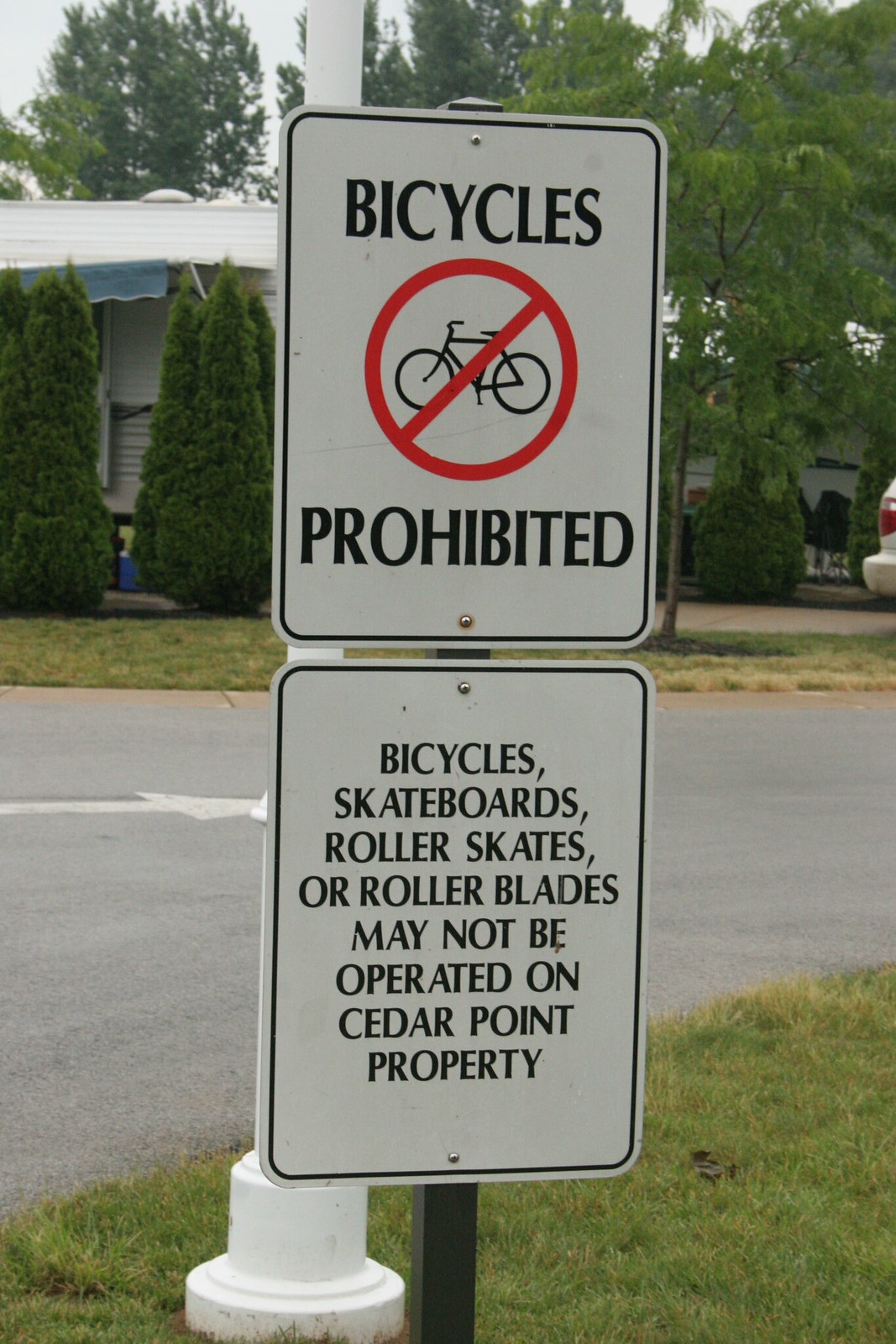This detailed photograph features a metal signpost with two rectangular, white metal signs positioned one above the other. The top sign, in big, bold black letters, reads "Bicycles Prohibited" and is accompanied by a red blocked-out symbol with a bicycle in the middle, indicating no bicycles allowed. The bottom sign, also in black font, states "Bicycles, Skateboards, Roller Skates, or Rollerblades may not be operated on Cedar Point property." Below the signpost sits a white fire hydrant, surrounded by a patch of green lawn. In the immediate background is a thick white light pole, behind which lies a paved street marked with a one-way arrow pointing to the right. Further back, manicured conical evergreen shrubs and additional trees can be seen, partially obscuring a house whose roofline is just visible.